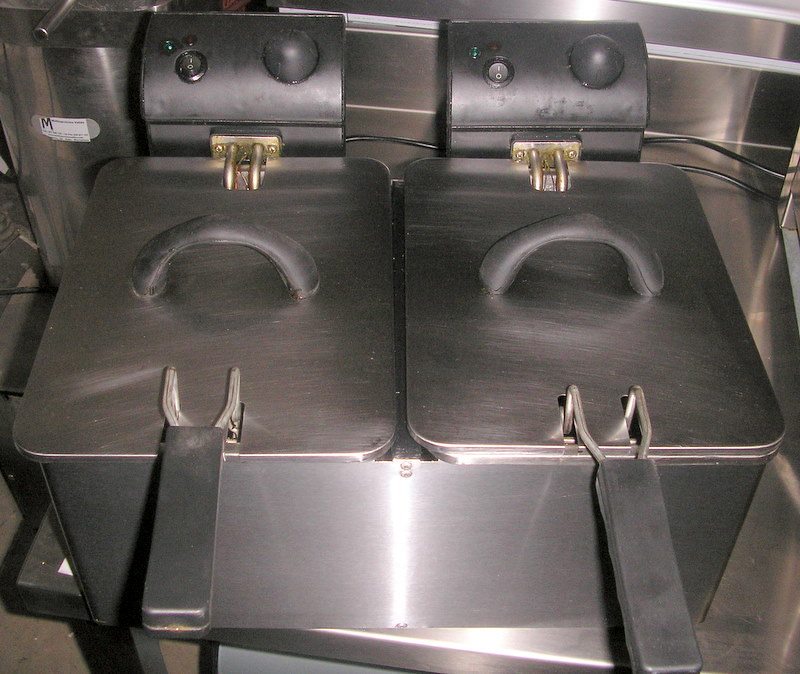The image depicts a double deep fryer, a large, industrial-grade stainless steel cooking apparatus designed for deep frying food. The rectangular machine features two separate compartments, each with its own lid. These lids are equipped with plastic handles on the edges and handlebar-like grips on top, which facilitate lifting and removal. Though the lids are closed, fry baskets appear to be inside, with their metal handles protruding through small holes in the front. The fryer includes a pressure valve and settings dial, indicating its functionality for pressure frying. The entire setup, which has a shiny yet deep metallic grey finish, is positioned on a steel table, with wires extending from the back, emphasizing its heavy-duty and industrial use.